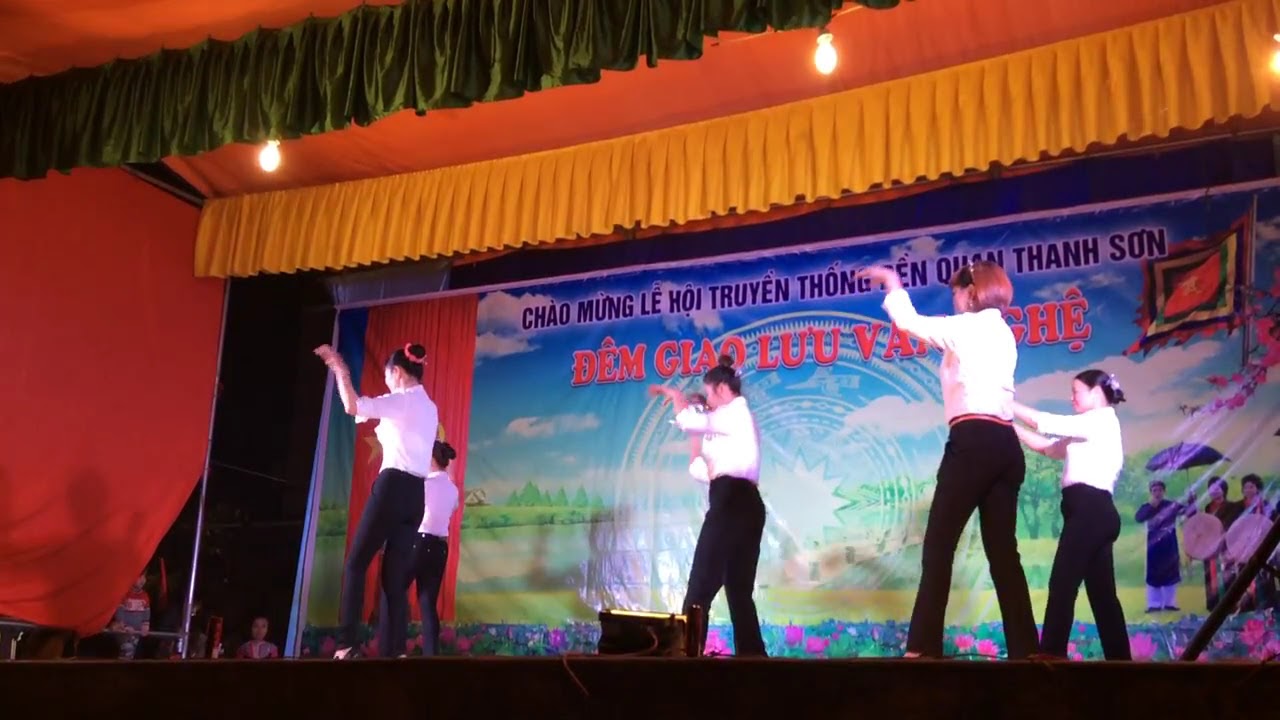The image captures a vibrant stage performance featuring five Asian women, each wearing white long-sleeved shirts and black dress pants. They are arranged in a scattered formation: two on the left, one in the center, and two on the right, with their hands raised in a pawing position and facing towards the left. The backdrop of the stage is adorned with a large, colorful banner displaying various Asian slogans in black and red letters. The text on the banner includes phrases like "Chao Mong Lai Hoi Chua Yen Thong" and "Dem, Jiao, Lu," though some words are obscured by the performers. The banner also features imagery of red, green, and bluish-violet plants and flowers, a starburst, a partly cloudy sky, and water—possibly a lake or river—surrounded by trees. The stage itself is rich with red and orange decorations, including fabric hanging from the ceiling and red walls. Spotlight fixtures and three visible light bulbs illuminate the scene. The perspective of the photograph suggests it was taken from the audience, slightly angled upwards. In the background, on the lower left corner, a female figure can be glimpsed standing behind the stage, suggesting the presence of other participants or crew members.